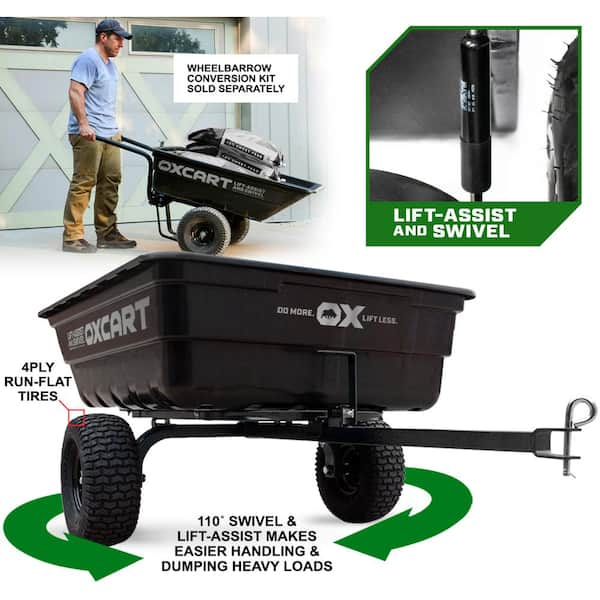The image appears to be part of an advertisement or instruction booklet for a black wheelbarrow called the Ox Cart. The top left features a photograph of a man wearing a baseball cap, a light blue shirt, and brownish pants, actively using the Ox Cart, which is loaded with several white cement bags displaying black writing. One notable section of the cart's black frame is highlighted with a close-up shot, bordered in green, indicating features such as "Lift and Assist" and "Swivel." 

The bottom section of the image focuses on the full Ox Cart against a white background, showcasing its robust design. The cart includes two thick, circular rubber tires described as "4-Ply Run Flat Tires" and an extension pole. Green arrows point out the "110-degree swivel" mechanism, emphasizing the cart's ease of handling and its capability for dumping heavy loads. Additionally, the bottom left corner mentions a "Wheelbarrow Conversion Kit," which is sold separately. The Ox Cart, with its slogan "Do More, Ox, Lift Less," promises enhanced functionality and efficiency for heavy lifting tasks.